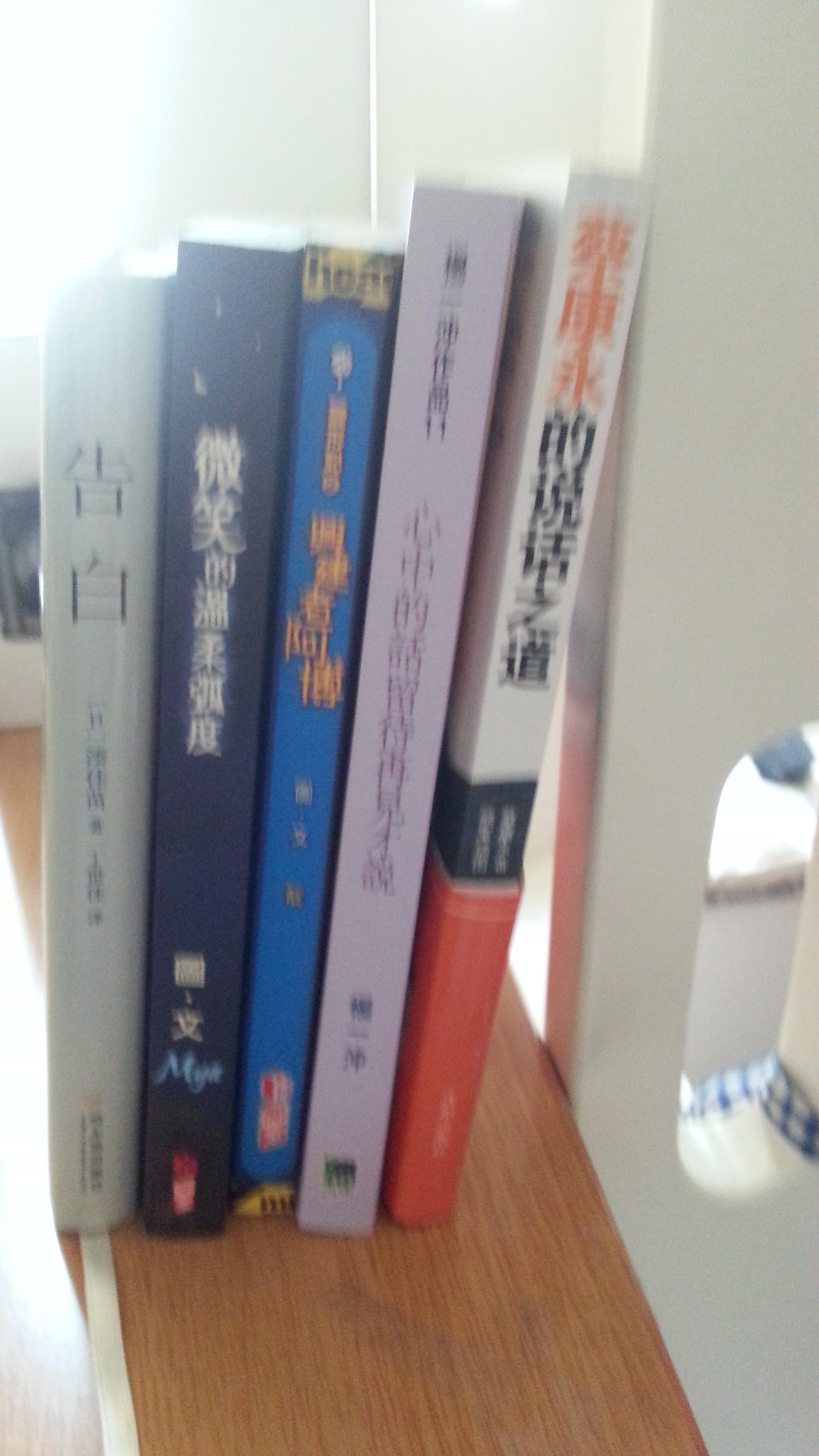This image features five books lined up on a wooden shelf, leaning slightly to the right against a white wall. The books have spines with Mandarin characters. From left to right, the colors are as follows: the first book is gray and has a white silk built-in bookmark peeking out from the top; the second book is black; the third book is blue with some yellow writing and a yellow bar across the top; the fourth book is mostly white with some purple writing, and the last book is the tallest, featuring a gradient from white at the top to black in the middle and red at the bottom. Bright sunlight shines from the top left corner of the image, creating a glare that slightly obscures the view. Alongside the books, there is a white element with a hole that stretches from the top to the bottom of the photograph, possibly part of the shelf or wall structure. Through this hole, one can glimpse a counter with a black object on it. The overall scene is tinged with the warmth of natural light, setting a calm and studious atmosphere.